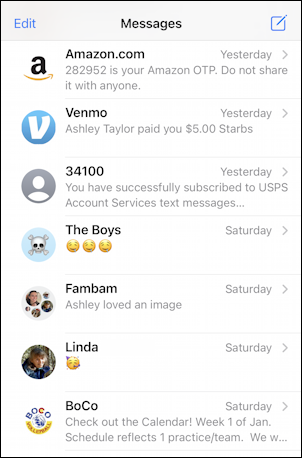The image is a screenshot of a message overview screen. In the top-left corner, a blue "Edit" button is displayed, while the word "Messages" appears prominently in black in the center of the header. On the top-right corner, there is a small box outline icon featuring a pencil.

The list of messages starts with:
1. A message from "Amazon.com," timestamped "Yesterday 20:29," which reads: "Your Amazon OTP is 52. Do not share it with anyone."
2. A message from "Venmo" indicating, "Ashley Taylor paid you $5."
3. A message from a number "34 100," stating: "You have successfully subscribed to USPS account services text messages."
4. A message simply labeled "The Boys," accompanied by three mouth-watering emojis.
5. A message from "Fam Bam," indicating, "Ashley loved an image."
6. A message from "Linda," who sent a celebration emoji.
7. The last message is from "Boco," which reads: "Check out the calendar. Week one in January schedule: Flex one practice team."